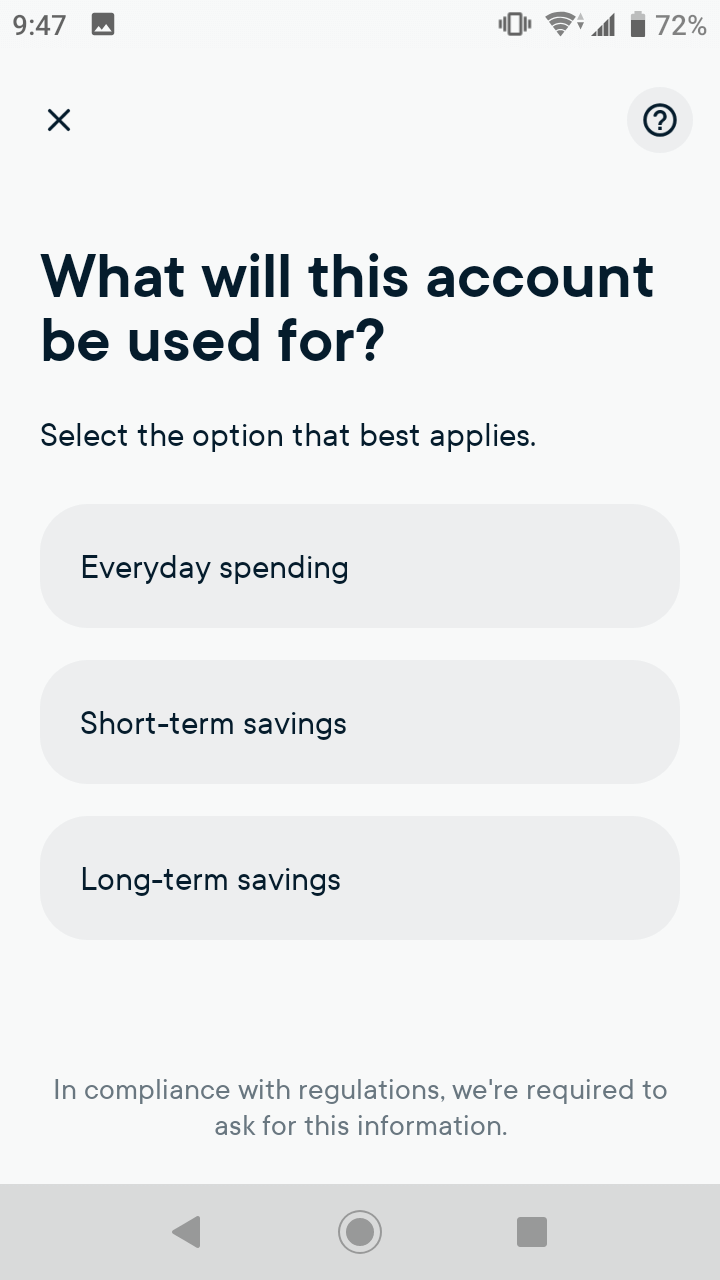This screenshot depicts a mobile application interface with a light gray background. At the top, the header displays vital system information: the time is 9:47 AM on the left, followed by an image icon. On the right, there is a phone icon indicating vibrate mode, a full Wi-Fi signal icon in dark gray, a full set of cellular bars, and a battery icon showing 72% charge with the percentage noted next to it.

Directly beneath this header is the main portion of the screen. In the top left corner, a black "X" icon allows users to close the screen. The top right corner features a light gray circle with a dark gray question mark inside, likely serving as a help or information button. 

Centered prominently in large black text is the question: "What will this account be used for? Select the option that best applies." Below this prompt are three selectable options, each within a light gray, pill-shaped box:
1. Everyday spending
2. Short-term savings
3. Long-term savings

The text on these options is in a thin serif font with only the first letter capitalized.

At the bottom of the light gray section of the screen, there is a disclaimer stating, "In compliance with regulations, we’re required to ask for this information."

Finally, the bottom of the screen contains a medium gray navigation bar featuring three icons: a solid gray circle with a thin, hollow circle around it on the left, a triangle with slightly rounded corners pointing left in the center, and a square with rounded corners on the right.